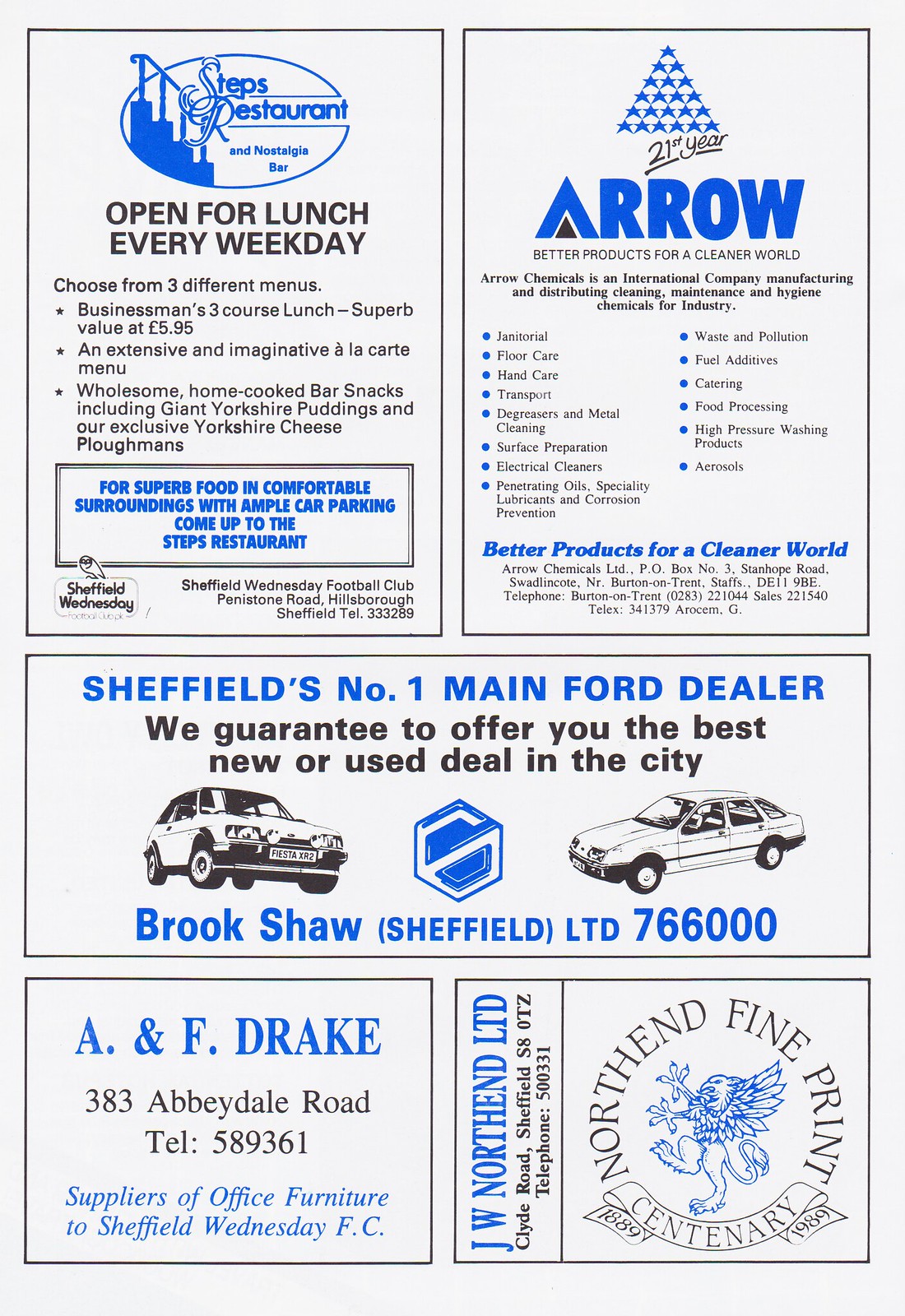This black-and-white page is filled with various advertisements, accented with some bright blue text and images. In the upper left corner, there's an ad for Steps Restaurant and Nostalgia Bar, which is open for lunch every weekday, highlighting the availability of three different menus. To the top right, Aero advertises its commitment to "better products for a cleaner world," explaining that Aero Chemicals is an international company specializing in the manufacturing and distribution of cleaning, maintenance, and hygiene chemicals for industry. Centrally located is the ad for Sheffield's number one main Ford dealer, which guarantees the best new and used car deals in the city and features two car illustrations. In the bottom left corner, there's an advertisement for A&F Drake, suppliers of office furniture. Finally, the bottom right corner features JW North End LTD, promoting Northern Fine Print with a centenary spanning from 1889 to 1989. This detailed flyer includes contact information for each business, making it a comprehensive resource possibly resembling something you'd find in a phone book or at the back of a magazine.